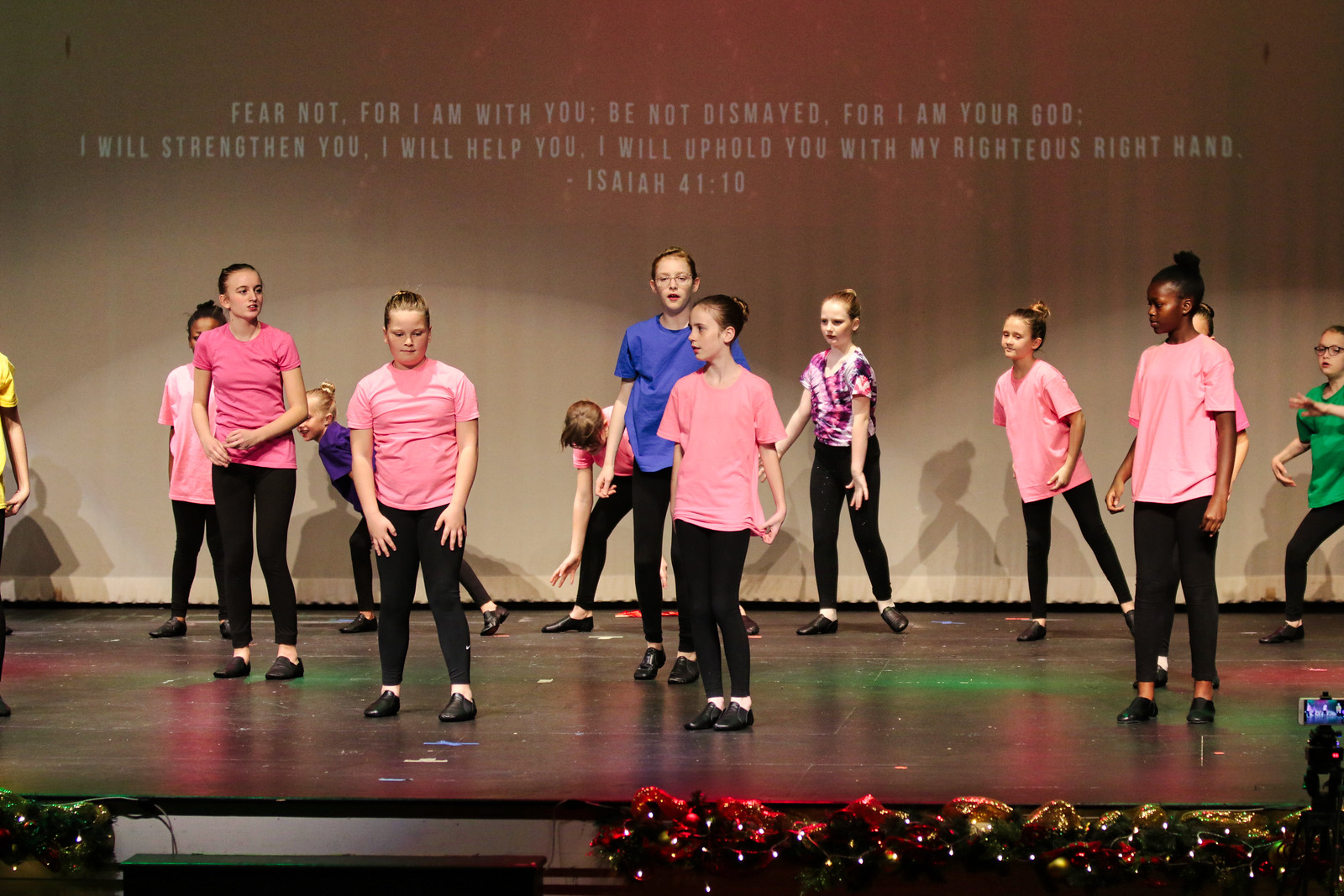The photograph captures a group of young girls, aged between 9 and 12, practicing on a decorated stage that appears to be set for a Christmas recital. The bottom edge of the stage is adorned with twinkling Christmas lights and festive ribbon. Most of the girls are dressed in pink tops, black leggings, and flat black shoes, though a few stand out in different colors: one in blue, another in green, a third in purple, and a glimpse of a girl in yellow on the left side. They seem to be rehearsing, as indicated by the taped spots on the floor and their casual attire. The back wall of the stage features a prominent biblical quote: “Fear not, for I am with you. Be not dismayed, for I am your God. I will strengthen you. I will help you. I will uphold you with my righteous right hand. Isaiah 41:10.” The scene suggests a moment of preparation and practice, likely addressing corrections or refining their routine under the guidance of their instructors.